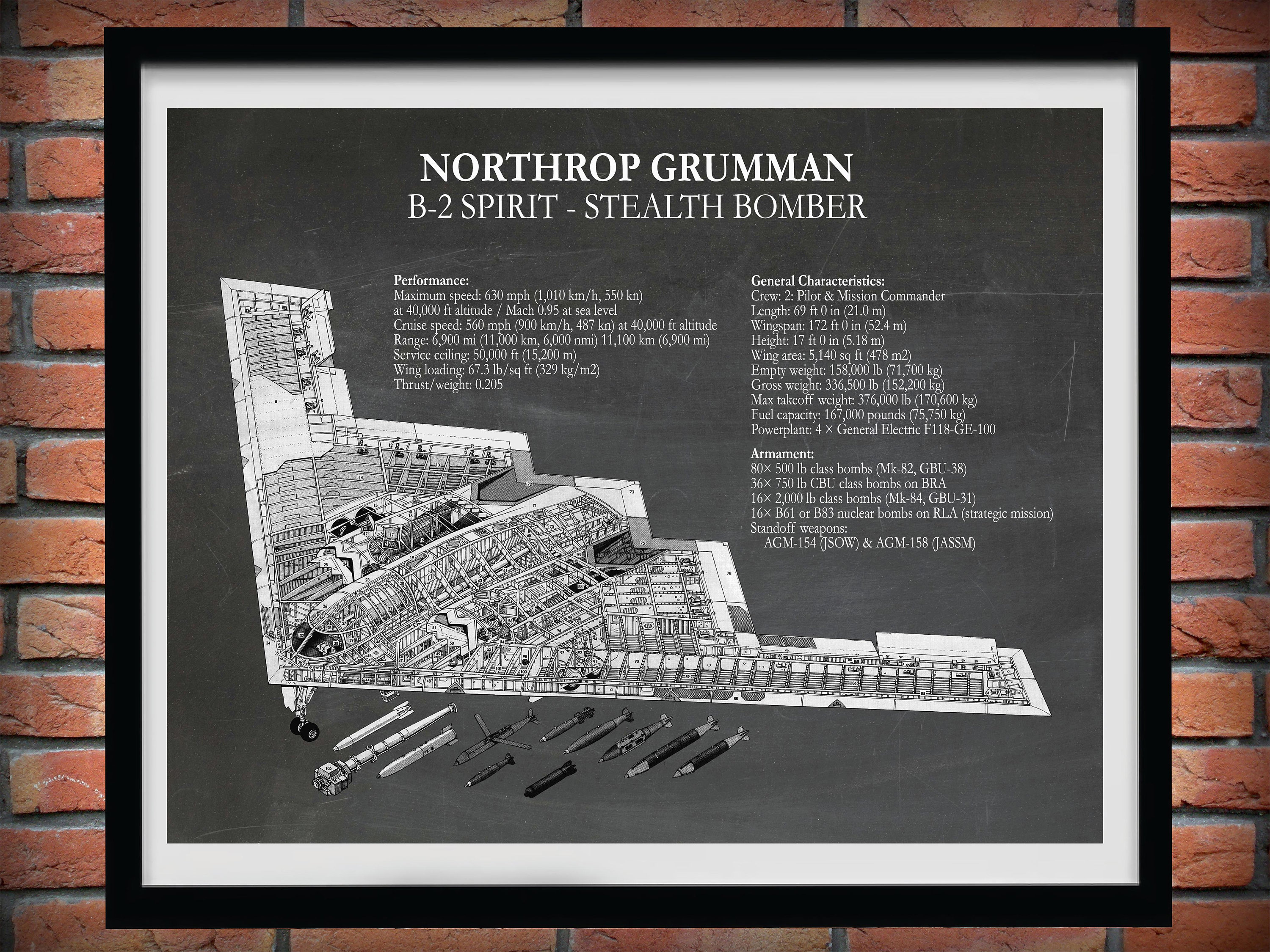Against a reddish-brown brick wall, a large, square-framed picture is displayed. The picture is encased first by a black border and then a white inner border. At the top of the image, white text on a gray background reads "Northrop Grumman B-2 Spirit Stealth Bomber." Below this heading, the picture features an intricate black-and-white diagram of the B-2 bomber, with a see-through illustration showing the bomber's internal components, including the missile arrangements, the wheels, and various internal mechanisms. Detailed specifications such as performance metrics—maximum speed of 630 miles per hour at 40,000 feet altitude, Mach 0.95 at sea level, a cruising speed of 560 mph, and a range of 6,900 miles—are listed alongside characteristics like the service ceiling of 50,000 feet and various thrust attributes. The armament section details the possible weaponry configurations of the bomber. Additionally, various metal components and images of potential armaments are shown beneath the main diagram, arranged in an L-shaped layout. The text throughout the image is detailed but may appear too small to read from a distance.